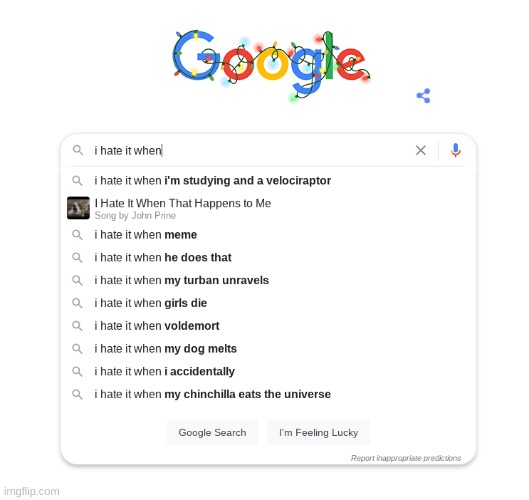The image depicts a festive Google homepage adorned with Christmas lights. The Google logo is presented in its iconic colorful format: a blue 'G,' a red 'O,' a yellow 'O,' a blue 'G,' a green 'L,' and a red 'E.' 

Near the logo, there's a small graphic of three interconnected circles symbolizing connectivity or linked ideas. 

In the search bar, the user has typed, "I hate it when," which auto-suggests a list of humorous and nonsensical completions, including:

1. "I hate it when I'm studying and have a velocipractor."
2. "I hate it when that happens to me," marked with an album cover related to a song by "John somebody."
3. "I hate it when Mimi."
4. "I hate it when he does that."
5. "I hate it when my turban unravels."
6. "I hate it when girls die."
7. "I hate it when Voldemort."
8. "I hate it when my dog melts."
9. "I hate it when I accidentally."
10. "I hate it when my chinchilla eats the universe."

These search suggestions highlight some quirky, inaccurate, and amusing entries. Each auto-suggestion is accompanied by a magnifying glass icon, suggesting they can be searched, except for the one related to the album cover.

Below the search bar are the familiar "Google Search" and "I'm Feeling Lucky" buttons. Outside of this interactive area, 'imgflip.com' is noted, likely indicating the source of the image.